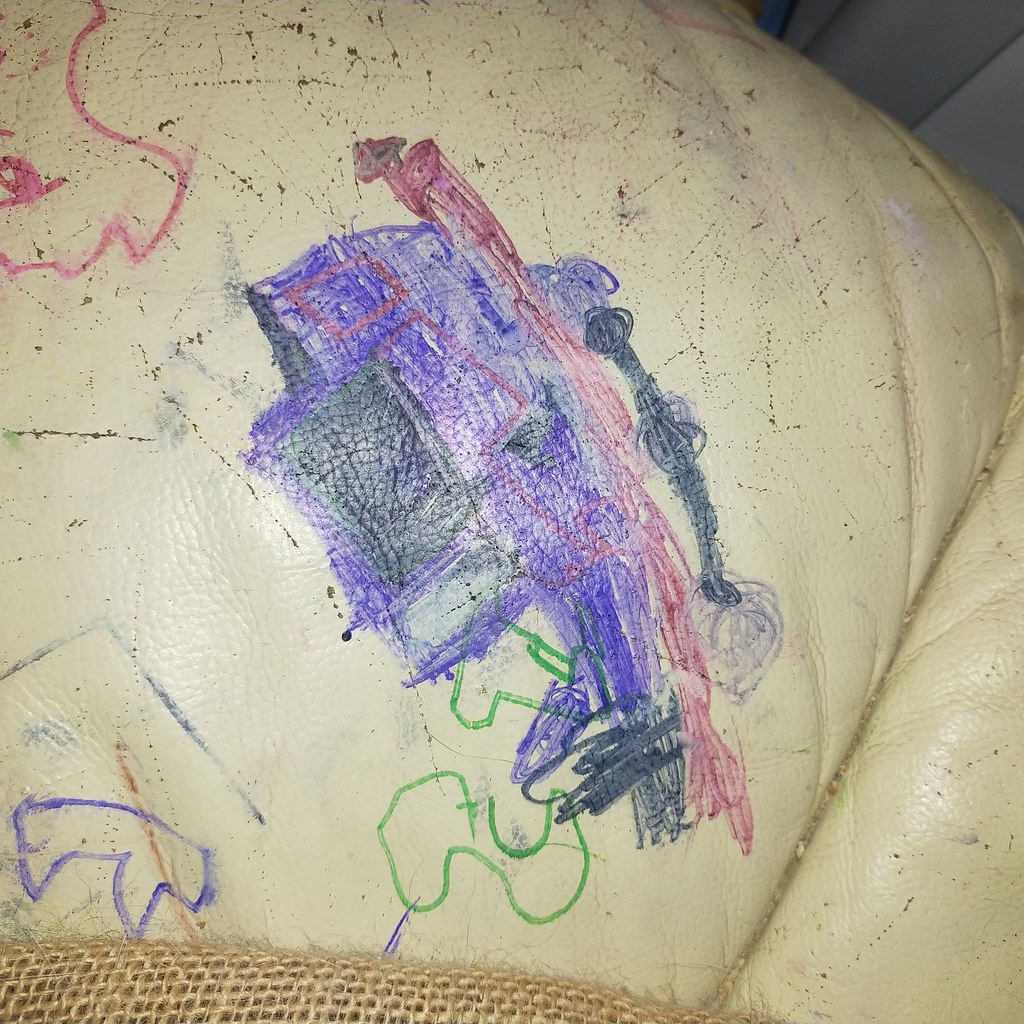In this image, there is a beige or tan leather couch, which is heavily marked with colorful crayon drawings. The scribbles include various shapes and vague depictions, possibly of a train or boat, executed in an array of colors such as green, blue, pink, and purple. The couch also features a netted rug draped over it, adding to the cluttered appearance. At the bottom of the photo, small pieces of debris or lint are visible, further suggesting a disorganized and playful atmosphere.